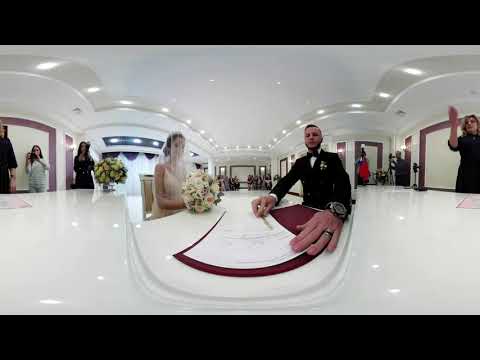In the photograph, a newlywed couple is seated at a gleaming white marble table in a grand, all-white hallway adorned with a series of ceiling lights. Central in the image, the bride, dressed in a traditional sleeveless white gown with a tiara and veil, holds a bouquet delicately placed on the table. Opposite her sits the groom in a black tuxedo with a flower in his lapel, a white shirt, a black tie, and a wedding ring with gold edges. He is focused on signing a document, likely the marriage license, with a black pen in hand.

Positioned at the marble table, the groom's serious demeanor contrasts with the celebratory atmosphere as guests are visible in the background. To the right, a woman appears to be holding out her hand, possibly asking questions to an unseen figure behind the camera. Behind them, two women film the proceedings, each equipped with video cameras. 

The hallway stretches extensively into the distance, with white walls, white floors, and brown wood trimmings framing sections of the wall. There is a hint of a window with curtains and a small flag hanging from a pole. Guests can be seen capturing the moment, some with cell phones. The entire composition conveys a moment of solemn commitment amid the joyous surroundings of what appears to be a beautifully appointed wedding venue.